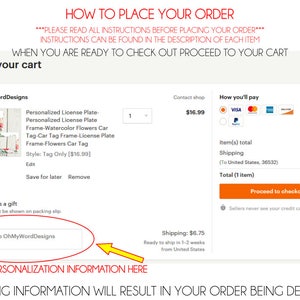**Detailed Caption:**

The image showcases a comprehensive order placement page with detailed instructions and relevant information. At the top of the page, highlighted in orange, are the words, "Order Placing Instruction on How to Place Your Order." Following this, three asterisks precede a bold orange instruction in capital letters: "Please Read All Instructions Before Placing Your Order," emphasizing the importance of understanding instructions provided for each item.

Beneath this notice, a gray bar prominently features the text "Your Cart" in bold black. Below, instructions in uppercase black letters direct users to proceed to their cart when ready to check out. 

The image includes a partially visible map and a section titled "Designs," featuring various personalized license plates and frames. Specifically listed is a "Personalized License Plate Frame Waterproof Flowers Car Tag," priced at $16.99, though the text is very small and difficult to read accurately. Options to edit, save for later, or remove the item are available via buttons next to the item details. Shipping costs are indicated at $6.75, with an estimated shipping time of one to two weeks, though some text is challenging to decipher.

A vertical gray line runs down the right side of the page, segmenting the payment information area. Payment options include Visa, MasterCard, American Express, Discover, and PayPal, with Visa currently selected. Information about the total items, shipping to the United States, and the total cost for one item is provided, alongside a zip code that is not fully legible. The "Proceed to Checkout" button is prominently displayed in orange with white text, accompanied by tiny, hard-to-read writing underneath.

To the left of the vertical gray line, there’s a designated area for personalization information marked with a circle and a yellow arrow pointing to the specified text box. This section lacks complete details as the words are cut off, ending abruptly with "information will result in your order being..."

The overall layout is cluttered and small text makes it challenging to read specific details clearly.